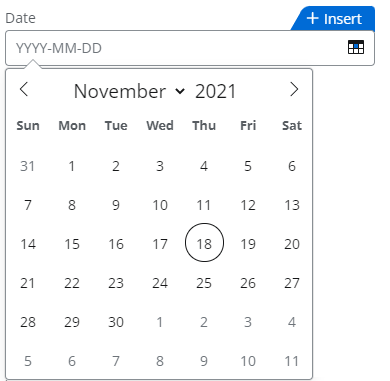The image depicts a user interface element for date selection. 

At the top left corner, there is a label displaying the word "Date." On the top right corner, a blue tab with white text contains a plus sign and the word "Insert." Directly below, a text box with a gray border is labeled "YYYY-MM-DD," indicating where to input the date. To the right of this text box, a small calendar icon is visible. This icon features a square with the top middle portion colored in blue and a black border at the top.

Beneath the text box, a dropdown menu extends downwards, displaying calendar options for year selection. The calendar interface is neatly enclosed in a white square with a gray border. At the top left corner of this dropdown, there is a left arrow, and in the middle, it displays "November" with a dropdown menu option, alongside "2021." To the right of this, another arrow points to the right. 

The calendar layout includes days of the week from Sunday to Saturday, listed from left to right. The month begins on a Monday, with the last day being the 30th, which falls on a Tuesday. The calendar also shows the last day of October and extends to display the first 11 days of December.